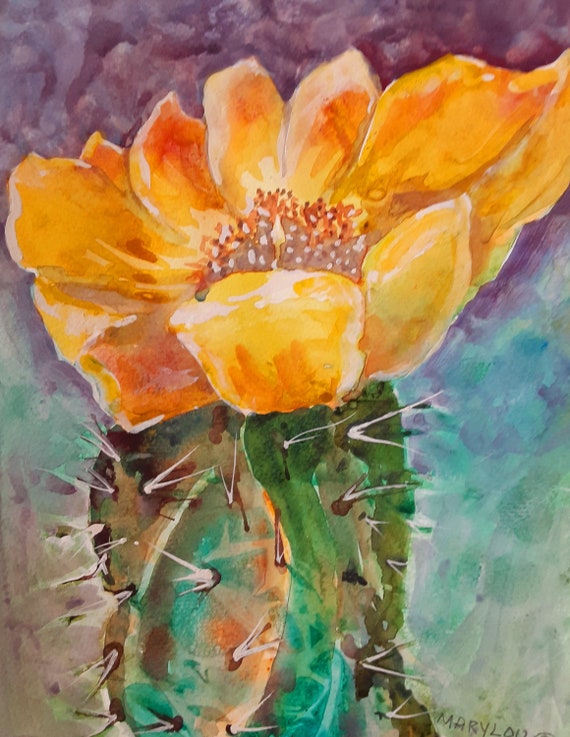This image showcases a vibrant painting of a cactus adorned with a blooming flower. The cactus, situated at the base, is depicted in various shades of green with noticeable white spikes. Emerging from the cactus is a striking flower, primarily in hues of orange and yellow, with its budding center beautifully detailed. Accompanying the flower at the top of the painting are additional small purple elements, enhancing its visual appeal. The background surrounding this central cactus is a blend of abstract colors, featuring blues, greens, and prominent purples, particularly towards the upper part of the image. The painter's signature, likely "Mary Lou," is partially visible in the bottom right corner, though slightly cut off. The vivid and harmonious combination of colors contributes to a calm and serene atmosphere, making this artwork not just a depiction of a cactus and its flower, but a sensory experience of tranquility and nature's beauty.